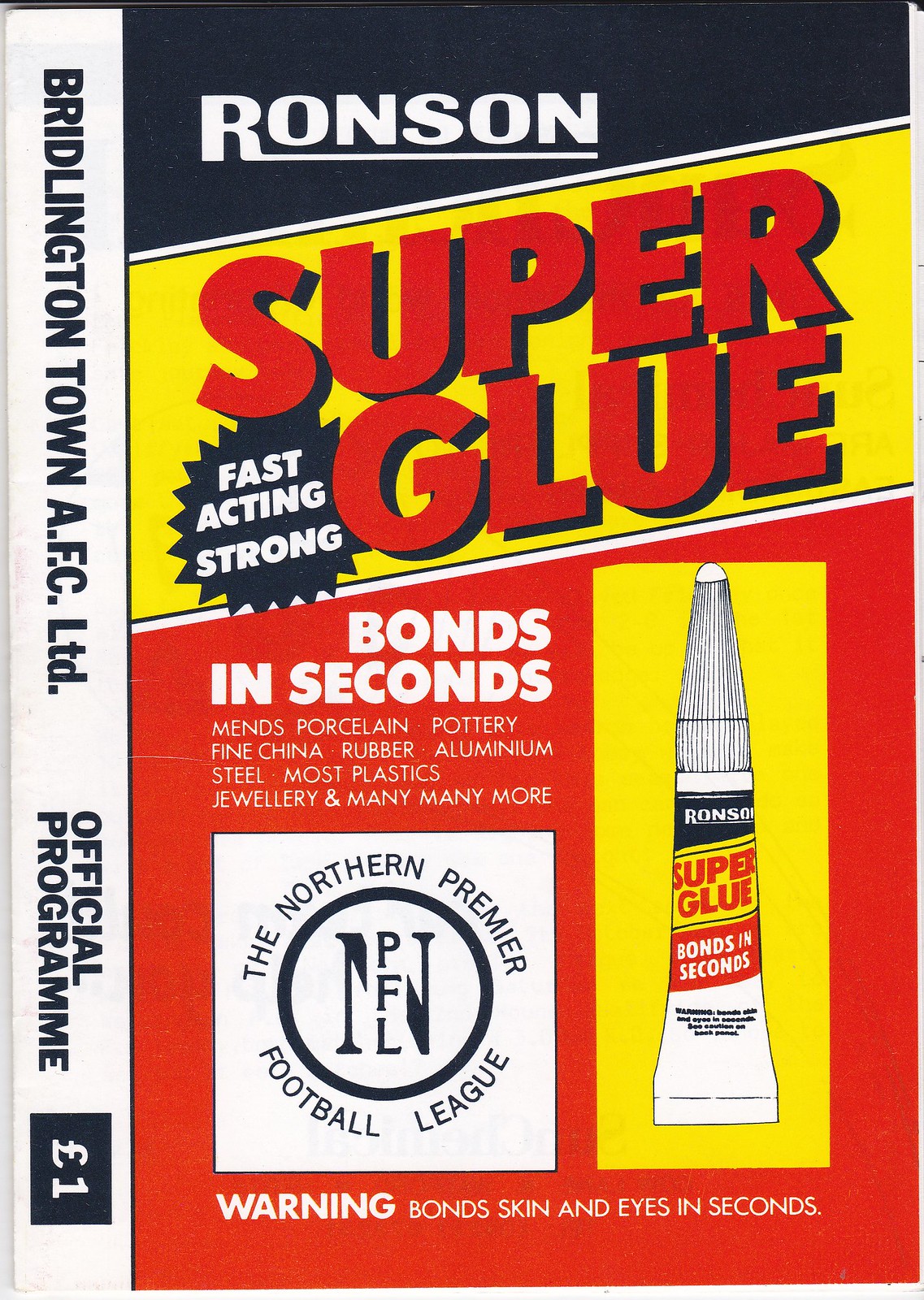The image is a vintage advertisement featured in a printed program for Bridlington Town AFC Limited, priced at one pound. The rectangular layout of the ad begins on the far left with a white background and sideways blue text that reads "Bridlington Town AFC Limited, official program, one pound." Beside it, a black banner with white text displays the brand name "Ronson." The center section of the ad has a yellow background with blue text proclaiming "Super Glue" and a small blue star with white text announcing "Fast Acting Strong." An artistic representation of a tube of Ronson Super Glue is prominently pictured against the yellow background. To its right, a red section bears the message "Bonds in Seconds" alongside the logo for the Northern Premier Football League, which is depicted with white background and blue print. Additional text details that the glue is effective for "men's porcelain, pottery, fine china, rubber, aluminum, steel, most plastics, jewelry, and many more." There is a warning at the bottom, stating "Bonds skin and eyes in seconds." The muted colors suggest the ad is from an older era, providing a nostalgic feel to the page.